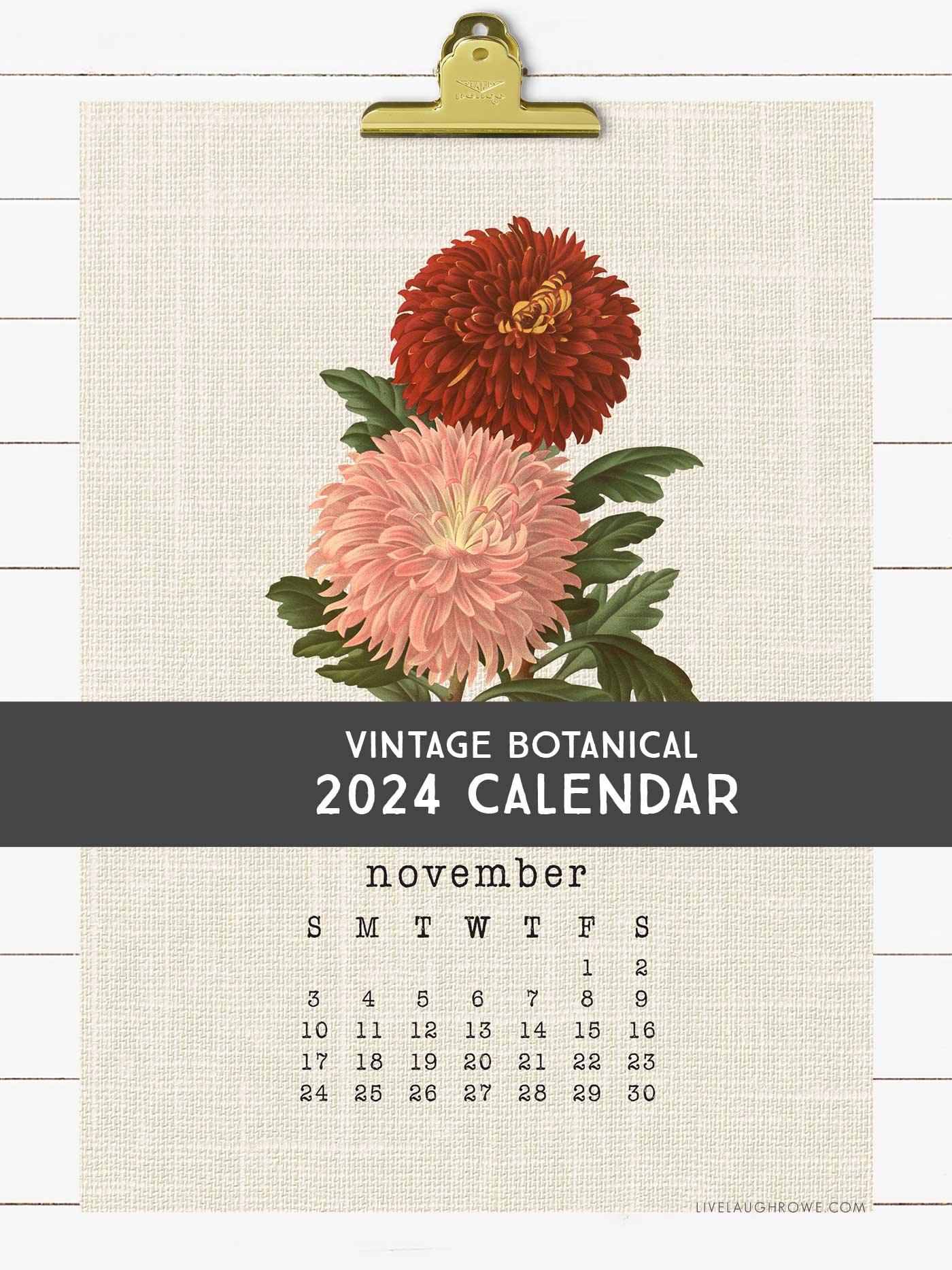This detailed photograph captures a vintage botanical 2024 calendar displayed on a white, horizontally paneled wooden wall. The calendar, held up by a gold clip reminiscent of a clipboard, features a piece of canvas-like paper as its main medium. Centered on this canvas are two detailed, spherical flowers—a maroon flower with an orangeish-red center at the top and a pink flower with a white center below it. The flowers are surrounded by lush, dark green leaves.

Directly beneath the floral illustration, a black rectangular bar spans the width of the canvas. Written in all-capital white sans-serif letters within this bar is the text "VINTAGE BOTANICAL 2024 CALENDAR." Below this title segment, the calendar displays "November" in lowercase, with the days of the week abbreviated as S, M, T, W, T, F, and S. These are followed by the dates arranged sequentially from 1 to 30.

Additionally, at the bottom right corner of the canvas, there is a website name "Live Laugh Row dot com," also in all capital letters, subtly incorporating a branding element into the overall vintage aesthetic of the calendar.